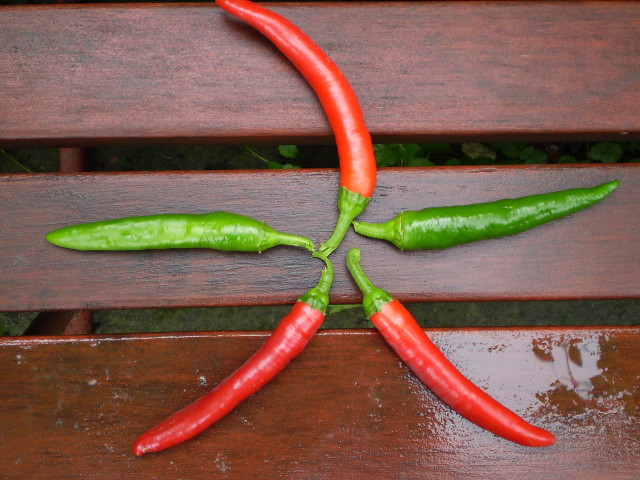This detailed color photograph, taken outdoors during the daytime, depicts a bench with a rich reddish-brown hue resembling mahogany wood. The bench is crafted from three horizontal slats, upon which five chili peppers are arranged in a star-shaped formation with their stems converging at the center. The star comprises three red peppers and two green ones. Specifically, a red pepper is positioned at the top, with a green pepper extending to the left and right, and two red peppers at the bottom left and bottom right. The peppers, slightly curved to the left, grow progressively larger as they extend outward from the center. The wooden surface appears to have a protective finish and shows signs of recent rainfall, evident from the water puddles visible in the bottom right corner of the image.